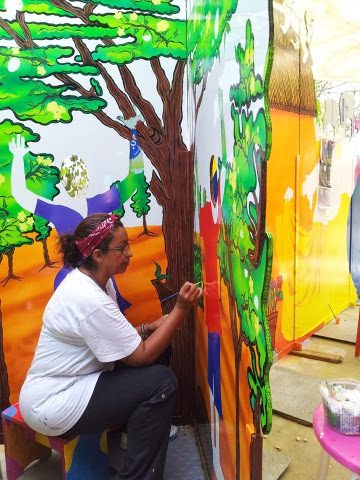In this captivating photograph, an artist is deeply immersed in the creation of a large and intricate mural that spans two connected walls. The artist, a woman with brown hair gathered into a ponytail and wearing glasses, is seen in profile from the right side. She dons a red and white bandana over her hair and a pair of earrings that catch the light as she focuses intently on her work.

Seated and holding a brush in her right hand, the artist is absorbed in painting with meticulous detail. On her left wrist, a bracelet glints subtly, complementing her white short-sleeved shirt and darker-colored pants. She appears to be in the final stages of her project, where most of the mural is already painted.

The mural itself is a vibrant, stylized depiction of nature embodying profound thematic elements. On one wall, a tree with lush leaves stands tall, alongside a figure depicted with arms raised. This character is rendered in an abstract manner where the face is a blend of natural elements, possibly leaves, in varying shades of green and yellowish-brown. The figure's right arm is a ghostly pale white, in stark contrast to the left arm, which melds hues of green, blue, and white. The torso, partially obscured by the artist's position, showcases a rich palette of blues and whites.

On the adjoining wall, the artist continues her nature-themed masterpiece. This section also features a bush and another human figure emerging under the artist's brush. This second figure is adorned in red clothing with blue shorts, and possesses strikingly bright white legs.

The photograph not only captures the artist at work but also the vibrant, dynamic essence of the evolving mural, a testament to her skill and creative vision.